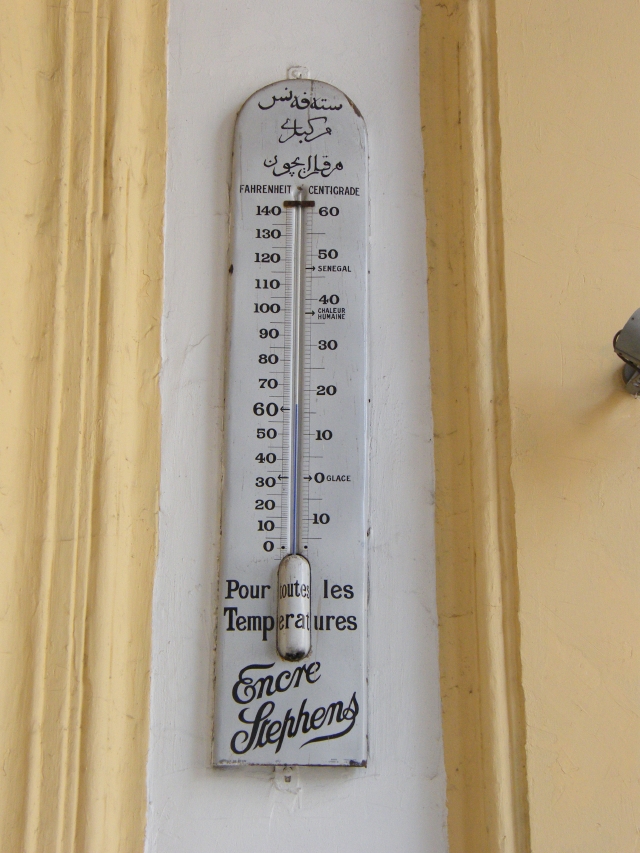The image showcases an antique alcohol thermometer mounted on a long, white metal strip with a curved top. The thermometer features a prominent bulb at the bottom, which is painted, obscuring its visibility. A dyed blue alcohol column runs through the capillary, indicating that it's not a mercury thermometer, which would appear silver. This thermometer is embedded into the flat metal strip, presumably for protection.

At the base of the thermometer, there is script text reading "Encre Stephens." Directly above that, across the bulb, are the French words "Pour toutes les températures," which translates to "For all temperatures." The thermometer displays both Fahrenheit and Centigrade scales. The Fahrenheit scale ranges from 0 to 140°F, and the Centigrade scale ranges approximately from -15 to +60°C.

On the Fahrenheit scale, 0 is labeled with the word "glace," meaning ice, denoting the freezing point of water. At 40°F, "chalure humaine" is marked, although its meaning is unclear in this context. Just below 50°F, the thermometer is marked with "Senegal," possibly indicating an extreme temperature recorded in Senegal, equating to around 47°C. At the top of the thermometer, there are three handwritten lines in Arabic.

The background consists of a white stucco or flat panel flanked by dark cream-colored woodwork, possibly part of a door frame. The intricate details and the bilingual temperature scales reflect the historical and geographical significance of the thermometer.